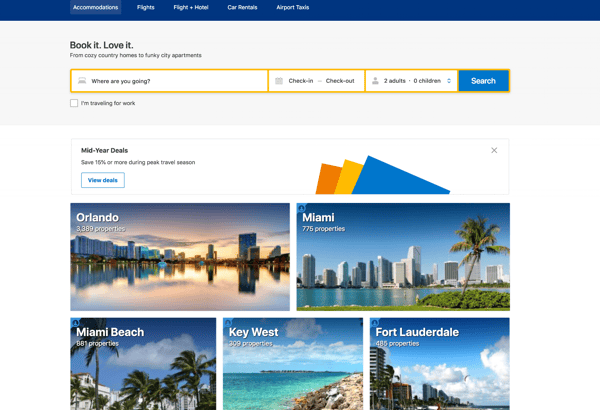This image features a dark blue header section with navigational options for "Accommodation," "Flight," "Flight + Hotel," "Car Rental," and "Airport Taxi." Beneath this, a light gray section contains the slogan, "Book it, love it, from cozy country home to funky city apartment." 

A gold-bordered bar follows, segmented into three white background areas, each with a blue "Search" button. The first segment prompts, "Where are you going?" The middle segment covers "Check In" and "Check Out" dates, while the third segment shows "Two adults, zero children." Additionally, there's a checkbox option labeled "I'm traveling for work."

Below this, an advertisement banner announces, "Mid-Year Deals: Save 10% or more during peak travel season," accompanied by a clickable button to view the deals. Further down, the image showcases five boxes, each displaying either a cityscape or a scenic beach. These boxes highlight popular destinations, naming Orlando, Miami, Miami Beach, Key West, and Fort Lauderdale.